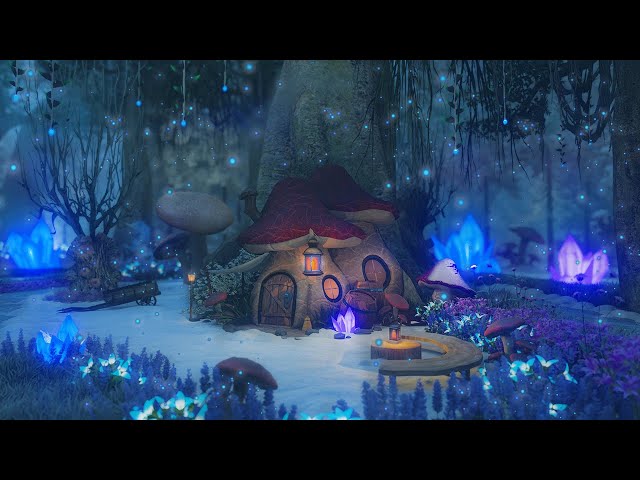The horizontal, rectangular drawing appears to be AI-generated and evokes a strong fantasy ambiance. The focal point is a small, enchanting mouse house crafted from two mushrooms, situated prominently in the center of the frame. The house features a wooden door and a lit lantern hanging from one mushroom, with circular windows adorning each of the mushroom caps. A chimney extends from one side of the structure. The mushrooms themselves are brown at the base, transitioning to dark red at the top. 

The entire scene is bathed in various shades of blue, punctuated by tiny, twinkling fairy lights that add an ethereal quality to the composition. Behind the mushroom house is a tall tree with long, draping vines. To the right of the house, a cozy semi-circle bench and a small round log serve as a sitting area, adorned with a tiny lantern. A wee mouse sits by an enchanting blue fire near the bench, surrounded by luminous foliage in blue and hints of pink.

The top eighth portion of the image is enveloped in darkness, with silhouettes of black trees adding a contrasting frame to the otherwise vibrant scene. Despite the cool color palette, the image exudes a warm, inviting atmosphere thanks to the meticulous details and enchanting light sources.